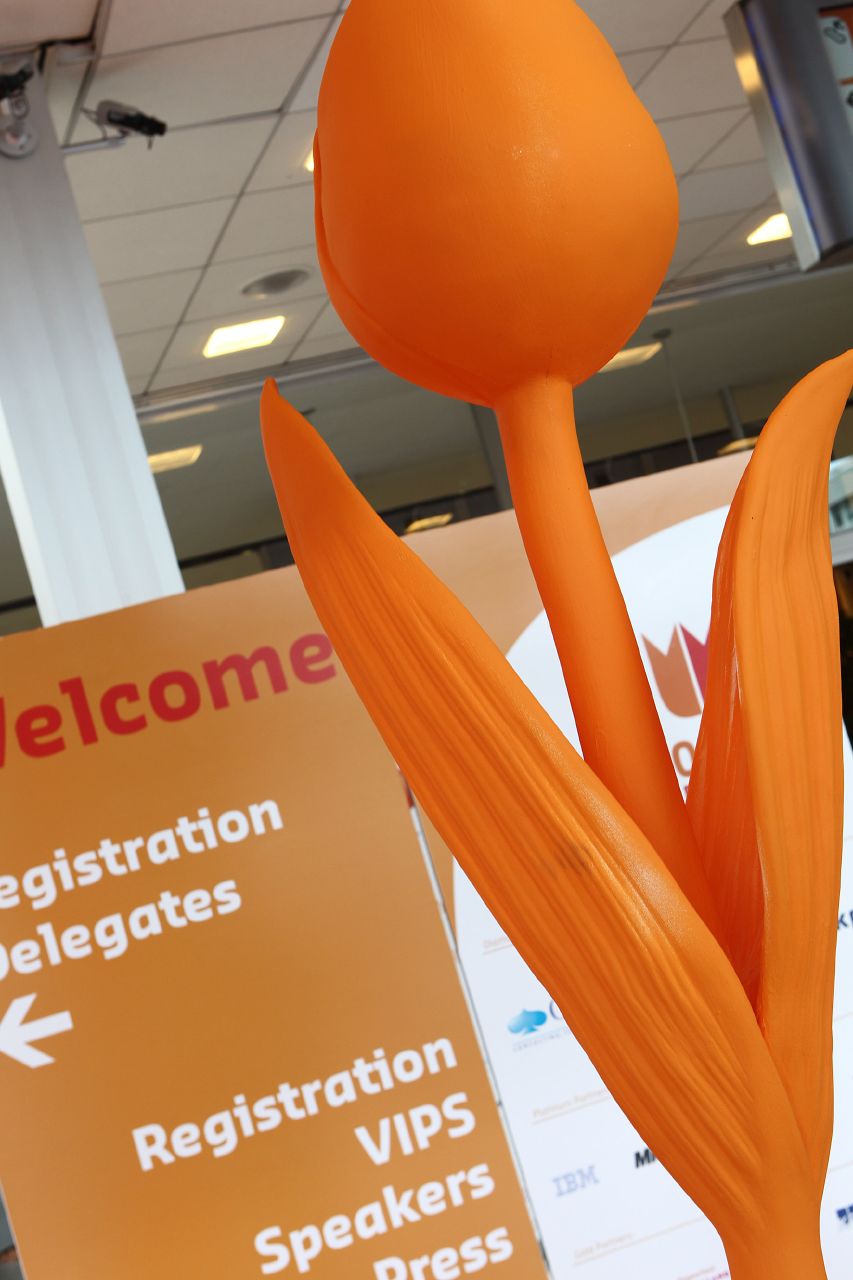This photograph, taken indoors, depicts a detailed scene primarily featuring a large, orange, artificial flower that appears to be 3D printed. The flower, complete with leaves and a stem, has a bulbous top and husk-like structures resembling corn. It is positioned in front of a sign, which seems to be part of a convention or event. The sign reads "WELCOME" in red letters on a light orange-tan background, and below it, partially visible text indicates directions for "registration delegates," "VIPs," "speakers," and "press," with an arrow pointing to the left. The image captures the ceiling made of white square tiles, illuminated by fluorescent lights. A CCTV camera is mounted on a pillar seen in the background. The photograph is slightly tilted to the left, adding a dynamic angle to the composition.